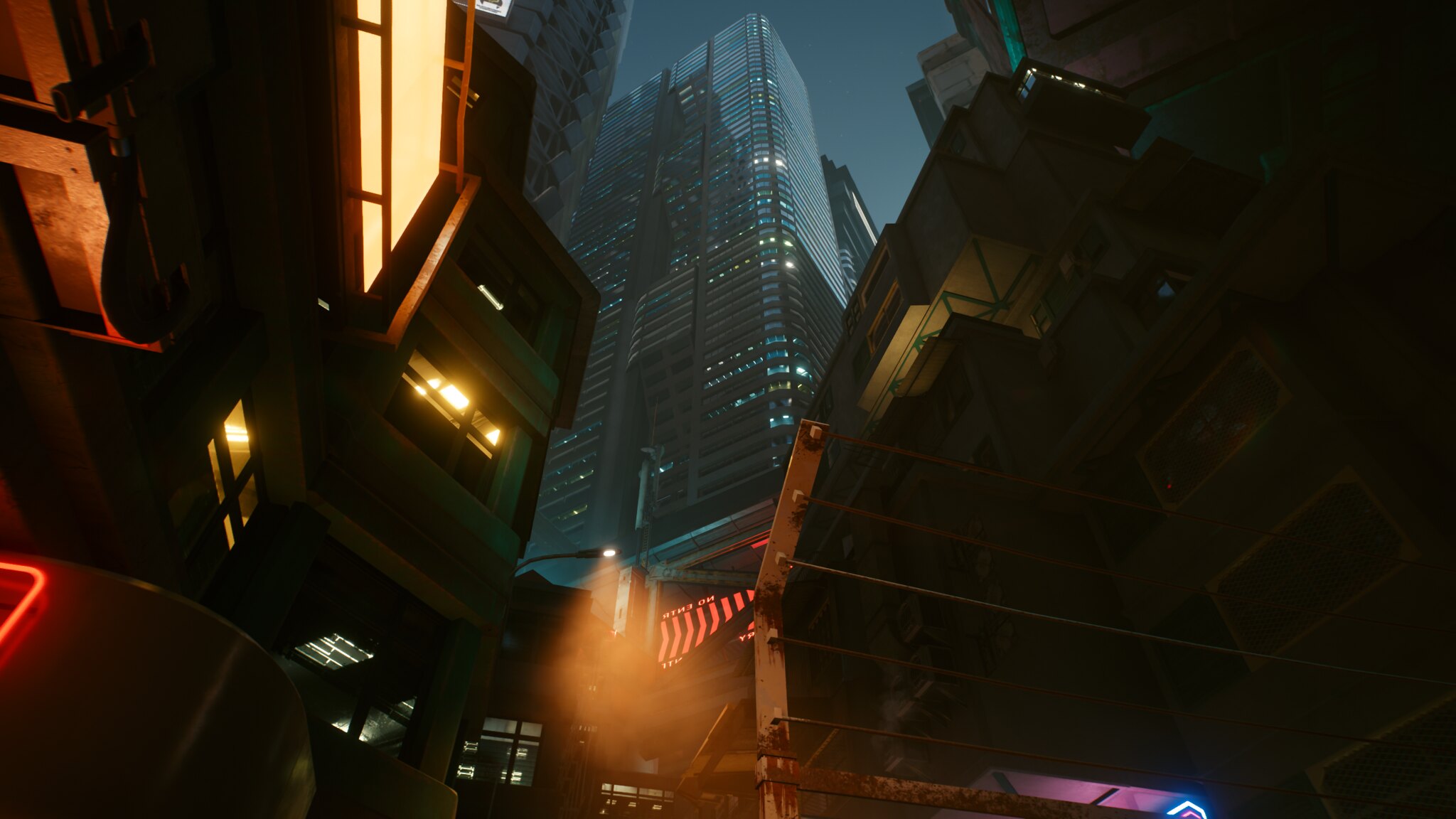This image appears to be a screenshot from the video game Cyberpunk 2077, depicting a cityscape from a street-level perspective. The scene is viewed looking upward at an angle, capturing the high-tech, neon-lit atmosphere of a futuristic urban setting. Dominating the center of the image is a large, silvery blue skyscraper with illuminated floors, framed by other tall buildings on the right and left. The foreground buildings feature various lights in their windows, glowing in vibrant oranges, golds, reds, and yellows against a backdrop of deep blue night sky. The neon lights and dark shadows create a striking contrast, emphasizing the cyberpunk aesthetic. Additional details, such as neon lights in the bottom right corner and possible doors in the background, further contribute to the immersive cityscape.